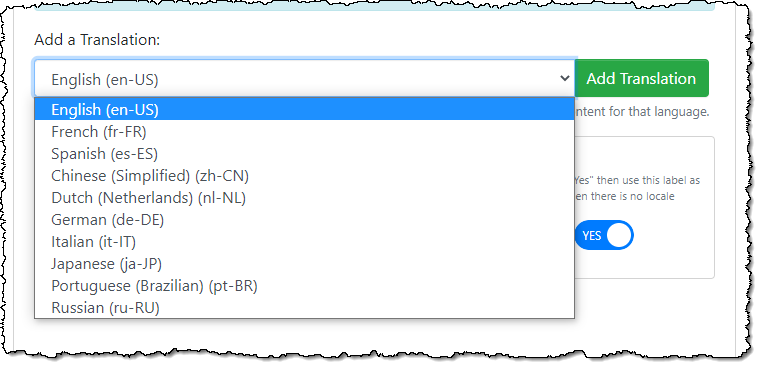The image appears to be a screenshot of a translation management software page, framed by a jagged black border that gives the impression it was torn from a book. The primary background color within this cutout is white.

At the upper section, slightly left of the center, there is a light blue square partly cropped out. Below this square, the text "Add a translation" is prominently displayed. Adjacent to this text, a dropdown menu has been activated, displaying several language options.

The first option in the dropdown menu is highlighted in blue, stating "English (en-US)." Following this, additional languages are listed in a similar format, each with a lowercase language code followed by an uppercase country code:
- French (fr-FR)
- Spanish (es-ES)
- Chinese (Simplified) (zh-CN)
- Dutch (nl-NL)
- German (de-DE)
- Italian (it-IT)
- Japanese (ja-JP)
- Portuguese (Brazilian) (pt-BR)
- Russian (ru-RU)

To the right of the dropdown, there is a green button with white text labeled "Add translation." Below this button, there is partially visible gray text that begins with "NTNT for that language," though it is cut off.

Further down the interface, there is a white box outlined in gray. Inside this box, it displays the text, "Yes then use this label as there is no locale." A blue slider switch is set to the "Yes" position, indicated by capital white letters on the slider.